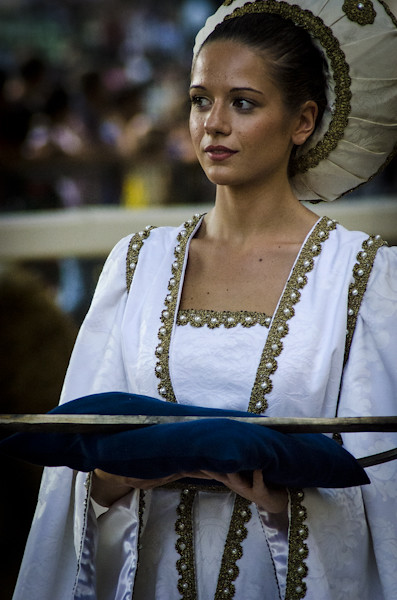This color photograph, presented in portrait orientation, captures a young woman in her 20s wearing medieval or religious attire, evocative of a reenactment or festival. She is attired in a flowing white gown adorned with green embroidery along the seams and fringes. The gown reveals a modest amount of her chest and is paired with a shroud or jacket that drapes over her shoulders, continuing the green embroidered theme. Her head is adorned with a distinctive puffy hat, resembling a medieval Pope's mitre or perhaps a pastry hat, adding an air of historical whimsy. The hat, which holds her hair back, is elaborately decorated with pleats and matching embroidery.

She has a tanned complexion, dark eyes, defined eyebrows, and red lips. Her expression is neutral as she gazes off to the right side of the image. In her hands, she cradles a rectangular silver tray or possibly a book on a stand, covered with dark blue velvet; the exact nature of the object is ambiguous due to its angle. The background features other people, but they are out of focus, ensuring that the primary focus remains on her detailed and ornate attire, fitting seamlessly into the photographic representational realism style.